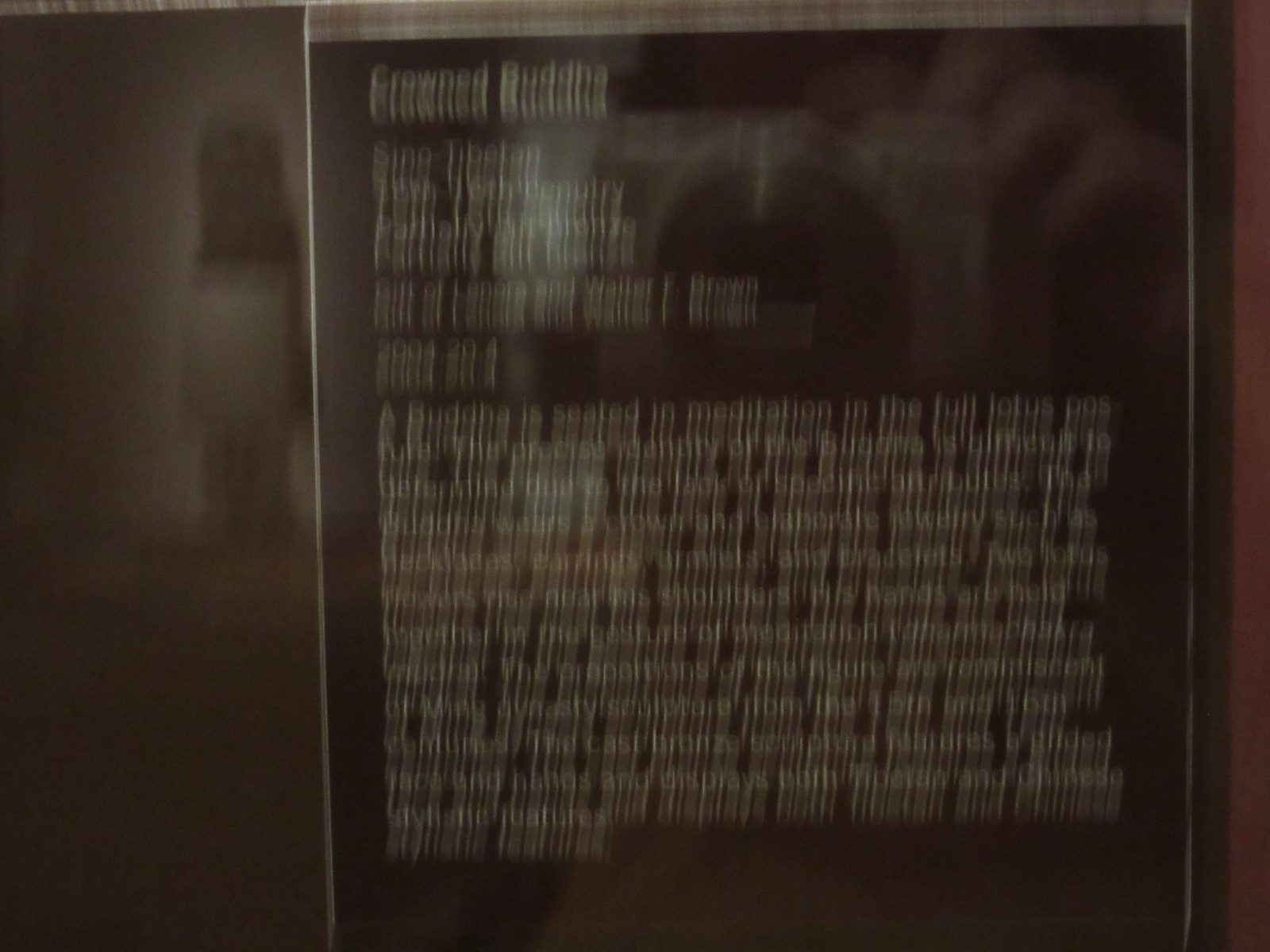The image is a blurred photograph capturing a descriptive plaque, presumably for an exhibit. At the top, partially legible text identifies the subject as a "Crowned Buddha" and mentions "Sino-Tibetan" origins. Below this heading, there is a large block of text that remains largely indecipherable due to the blur, but fragments suggest it describes a Buddha seated in meditation in the full lotus position. The photograph also reflects a person holding a camera, evident from a hand seen clutching the device. In the background, partially visible through the reflective glass, is a black statue with a white center, likely the statue being described by the text.